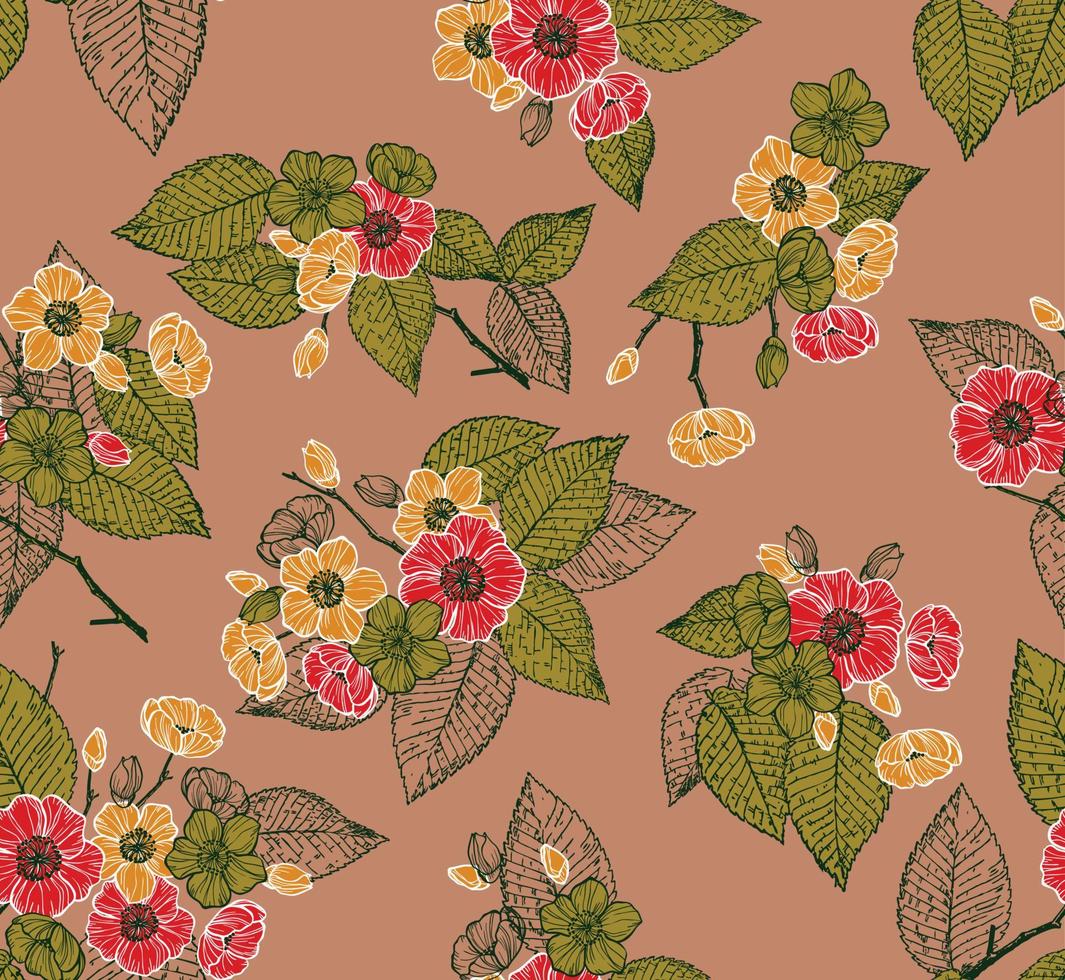This image features a detailed illustration that could be a wallpaper or fabric pattern. The background is a soft blush mauve hue, providing a subtle and elegant backdrop. Scattered throughout are floral clusters, each containing a mix of both colored and monochrome elements. The clusters consist of small round red and yellow flowers, with the yellow ones having distinct black centers. Green leaves accompany these florals, some fully colored in and others rendered as clear, skeletonized outlines. There are approximately ten full and partial clusters, each presenting a combination of vibrant colors and simple, black and white outlines. This repetition of elements creates a harmonious and thoughtful design, where every bouquet consists of varying stages of bloom, from closed buds to fully opened flowers.